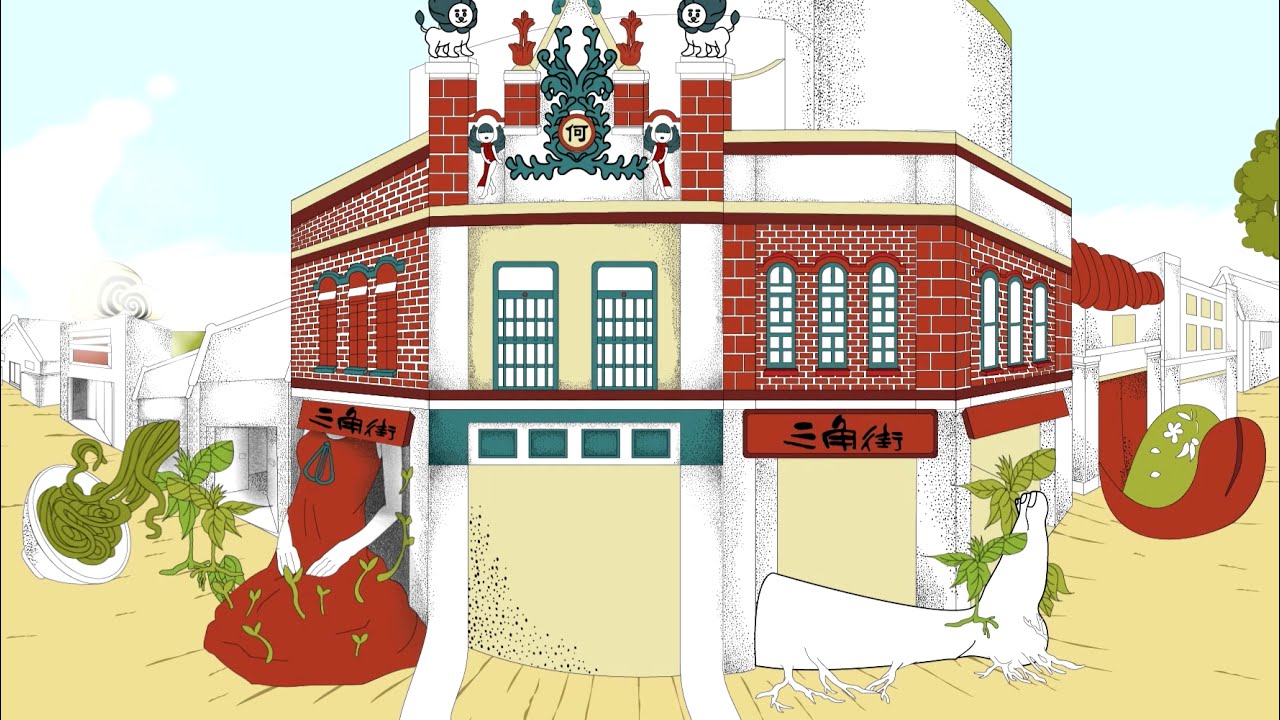The image depicts a quirky cartoon or computer-generated scene of a multi-story building with an eclectic and festive design. The building appears slightly curved, almost hexagonal, featuring a mix of white concrete, red and white brick, and stucco. The house is adorned in yellow, green, and red hues, complemented by teal-framed windows and red arches. The top floor boasts a greenish-blue scroll with a circle containing an emblem or possibly an Asian character, flanked by two lion statues that have white faces with similar characters.

The scene incorporates holiday decorations, with wreaths or English-style emblems and holly scattered abundantly around. Stockings in green and red colors lean against the house's side, adding to the festive atmosphere. Interestingly, the bottom part of a woman in a red dress with plants growing out of her is visible on the left side of the image. A solid white foot emanating from the right wall has veins or roots reaching into the ground, interspersed with plant life.

To the far right, a red tongue emerges from the building, curving around a green object adorned with white flowers and leaves. Nearby, the head and neck of a horse with greenery around its mouth are visible. The scene is set against a backdrop of a blue sky with small, fluffy white clouds.